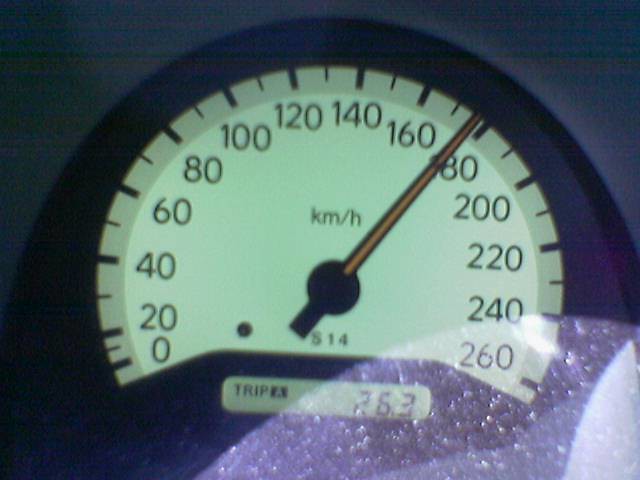The image depicts a speedometer, typically found in a car, with a design resembling a clock face. The speedometer displays a measurement range from 20 to 260 kilometers per hour, marked in increments of 20 (20, 40, 60, etc.). The numbers are arranged in a near-complete circle around the edge of the dial. In the center, the abbreviation "KM/H" signifies kilometers per hour.

A needle, or pointer, is currently indicating a speed close to 180 km/h. The background of the speedometer is a glowing green hue, making the markings and numbers stand out clearly.

At the bottom of the speedometer display, the text "Trip A" is visible, accompanied by the number 26.3, which likely refers to the distance traveled in kilometers on a specific trip. Below the needle, the characters "S14" are shown, though their exact meaning is unclear.